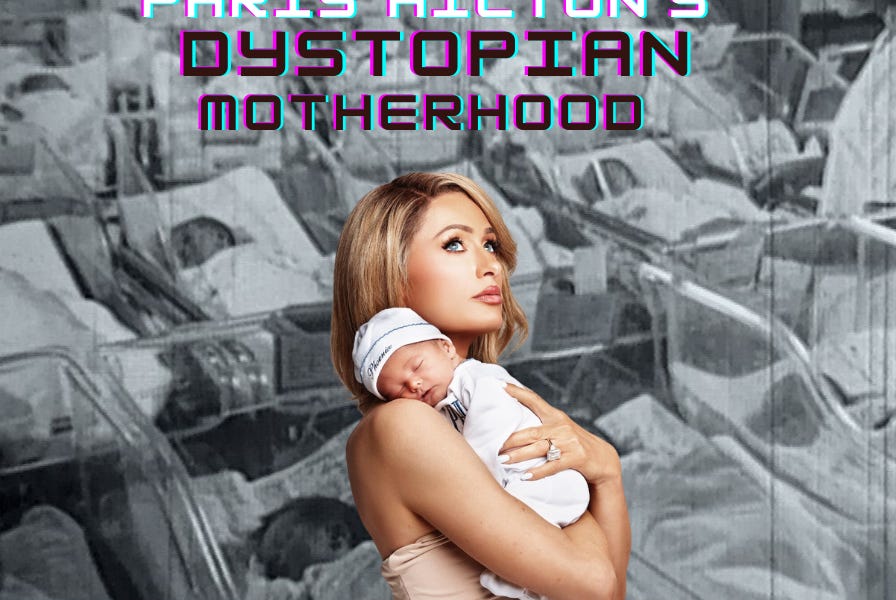The image depicts a modern color photograph of Paris Hilton, dressed in a strapless, tan-colored top with blonde hair cascading over her shoulders. She's holding her infant child, who is wearing a white onesie with blue accents and a white hat featuring blue text and trim. The baby rests on her right shoulder, with Paris's hand gently supporting the child. Prominently, Paris is adorned with a large ring on her ring finger, indicating she is married. The background contrasts sharply as it is a black and white, vintage-style photograph depicting numerous newborns in clear hospital incubators, lined with gray and white blankets. A nurse stands to the right among the rows of infants. Adding to the striking depiction, the top of the image features the text "Paris Hilton's Dystopian Motherhood," capitalized in black lettering with blue and purple outlines, merging the contemporary and nostalgic elements of the photograph.